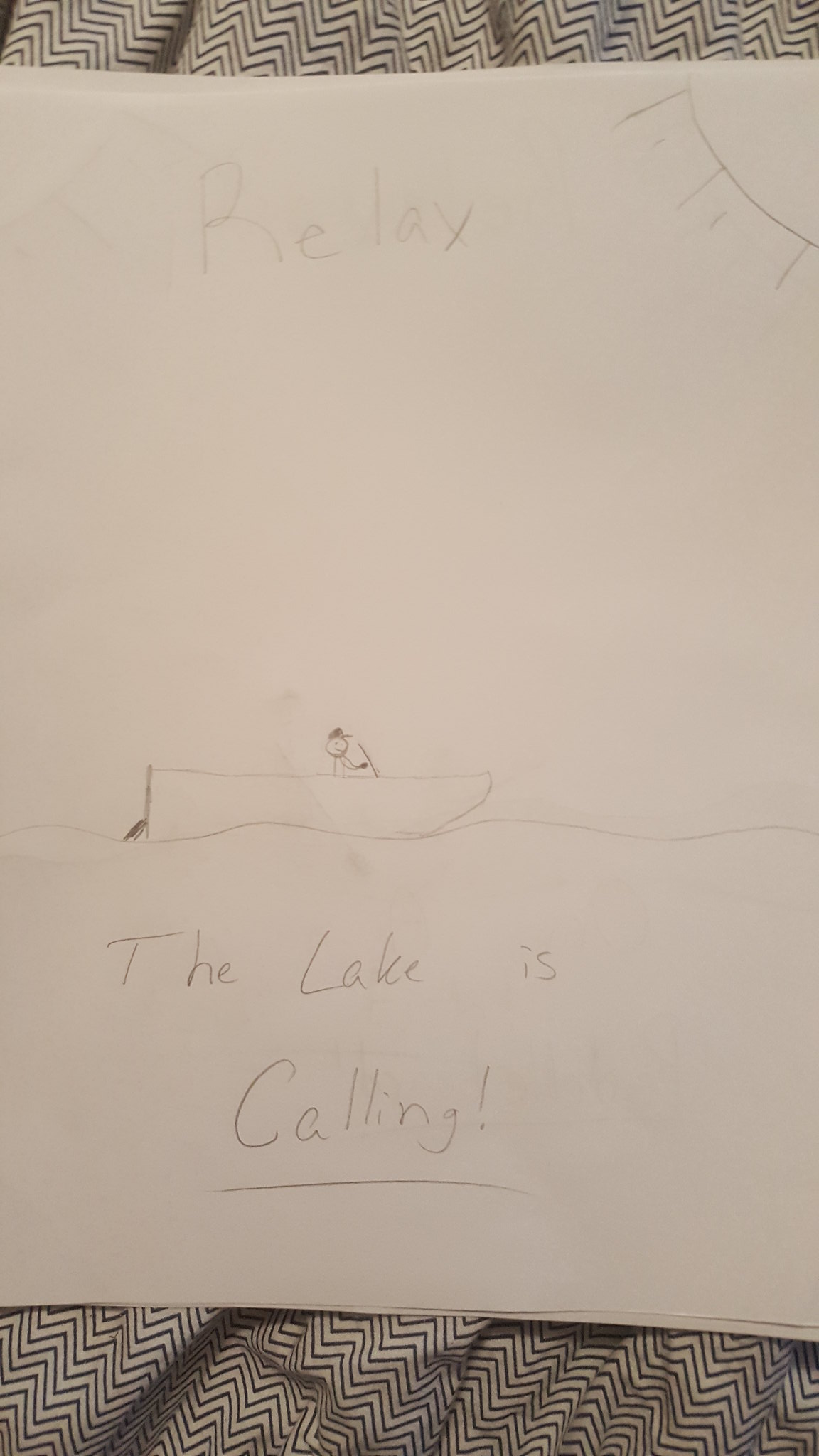A white piece of paper rests on a brown and white herringbone-patterned tablecloth. At the top of the paper, written in very light pencil, is the word "Relax." In the top right-hand corner, there's a partial sketch of what seems to be a sun, depicted as an oval with small lines radiating outward. Beneath the word "Relax," there is a simplistic drawing of a boat with a small round head inside, possibly representing a person holding the steering wheel. Below the drawing, the phrase "The lake is calling!" is written, with an exclamation point emphasizing the word "calling."